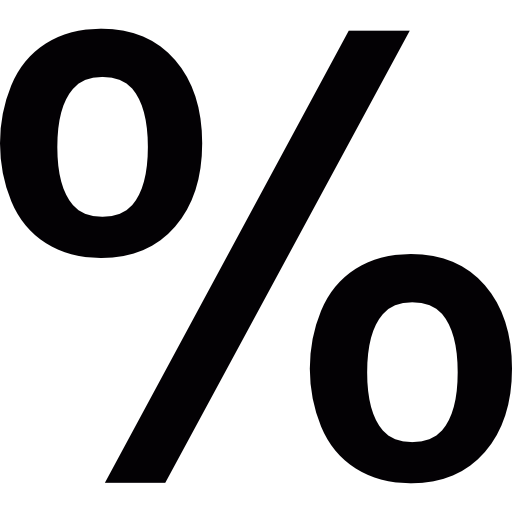The image is a striking black and white graphic design of a percent sign (%). It features a large black circular zero positioned in the top left corner and a similarly sized black circular zero in the bottom right corner, both filled with white. Connecting these two zeros is a bold, black, forward-slash line that diagonally traverses from the bottom left to the top right. The background of the image is a stark, plain white, enhancing the contrast of the percent sign elements. The design appears computer-generated with precise, clean edges, emphasizing its modern, minimalist aesthetic.